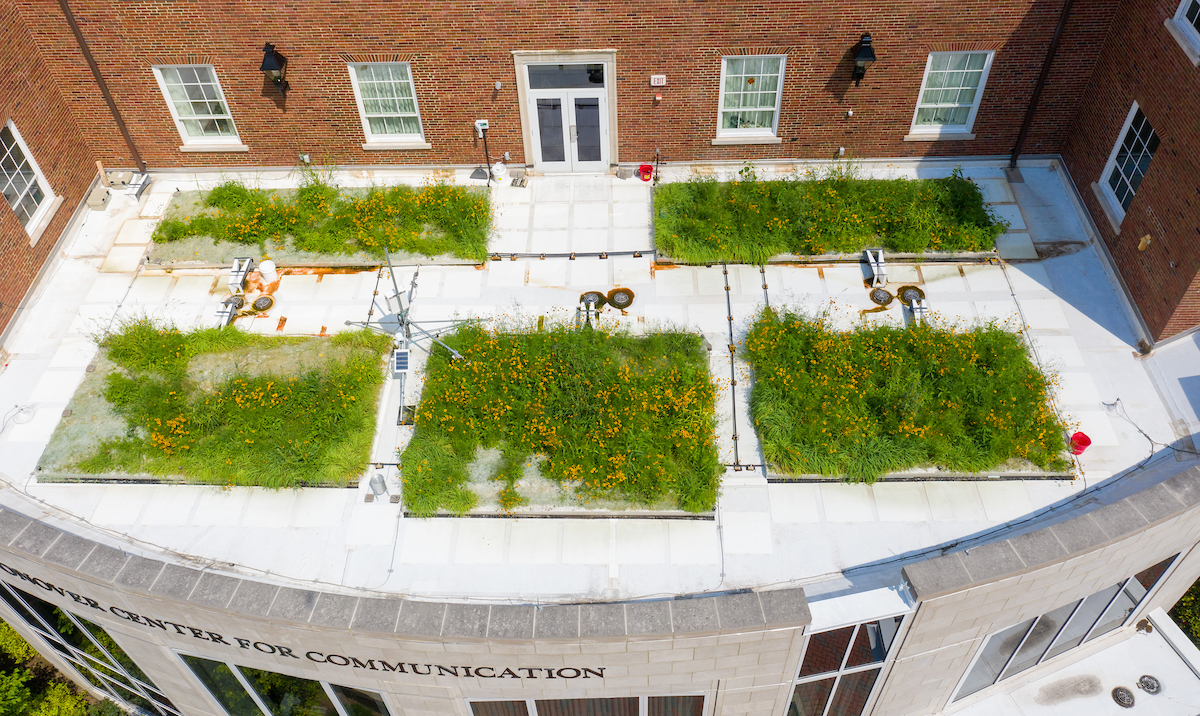This aerial photograph, likely taken by a drone, captures the rooftop of a modern brick building, identified partially by its inscription as the "Center for Communication." The roof, predominantly flat and white, features five rectangular garden beds planted with grasses and wildflowers, possibly including dandelions. Various devices, potentially for measurement or communication, are situated around the garden beds, adding to the unique rooftop landscape. The building's roof is accessible via double glass doors flanked by two large black sconce lights and additional windows, all part of the structure's L-shaped extension.